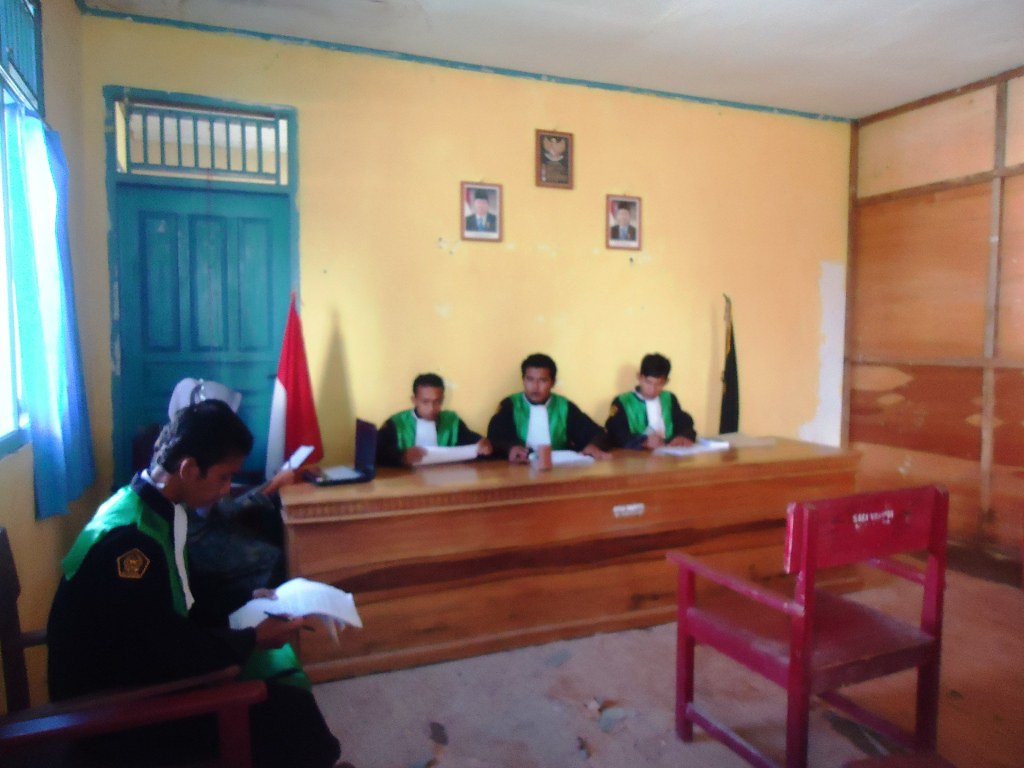In this photograph, taken perhaps in Mexico inside a government building, four gentlemen clothed in black and green uniforms appear engaged in official duties. The three men seated behind a wooden desk are flanked by a red and white flag on one side and a black flag on the other. The fourth man, positioned on the lower left corner of the image, sits reading a piece of paper. An empty red chair is prominently placed in front of the desk. Behind the men, the yellow wall, adorned with three photographs, contrasts with the brown elements in the room and the blue door visible on the left side. The entire scene captures a moment of local government officials diligently reviewing documents.